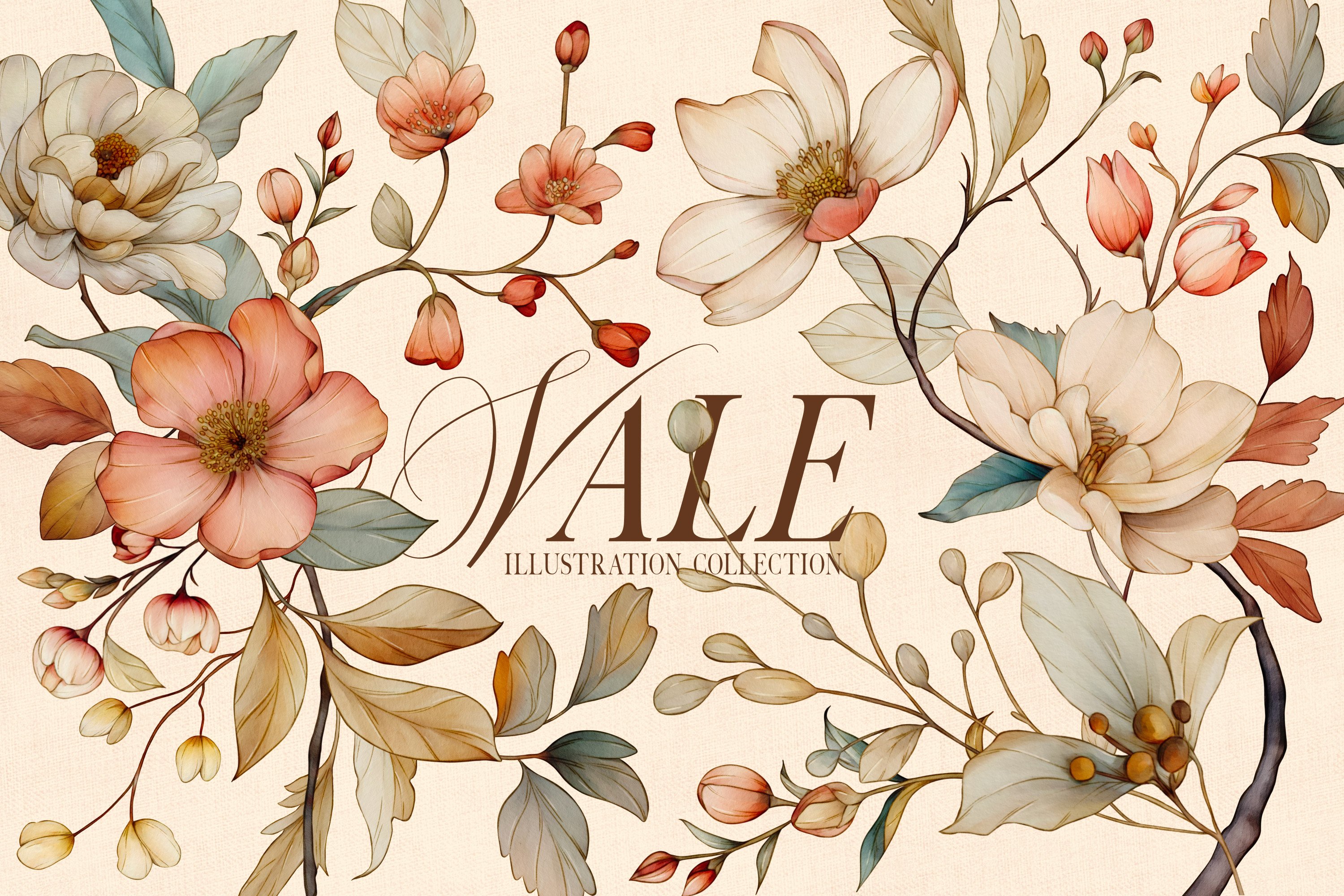This digital art illustration features an intricate array of flowers and leaves, meticulously depicted in an elegant and delicate style. Central to the artwork is the bold text "VEIL ILLUSTRATION COLLECTION," written in stylized dark brown capital letters with a uniquely designed "V" in "Veil." The flowers display a spectrum of soft colors, including red, pink, cream, pale orange, and white, with vibrant yellow centers. Among these flowers, some are fully bloomed while others remain as buds, contributing to the diversity of the scene.

The leaves accompanying these floral elements come in various shades including blue, brown, beige, and rose, creating a harmonious blend. Two main stems extend from the lower corners of the image—one from the bottom left extending upwards and another from the bottom right, also growing upwards. From these stems sprout the branches that hold the flowers and leaves, adding structure to the delicate composition.

Set against a light, pastel pink background, this artwork exudes a gentle and inviting atmosphere, further emphasized by the soft hues and intricate details. The "VEIL ILLUSTRATION COLLECTION" text in the center suggests a curated collection of floral illustrations, inviting viewers to explore beyond the initial image. The overall presentation, with its blend of colors and forms, captures the essence of natural beauty and delicate artistry.